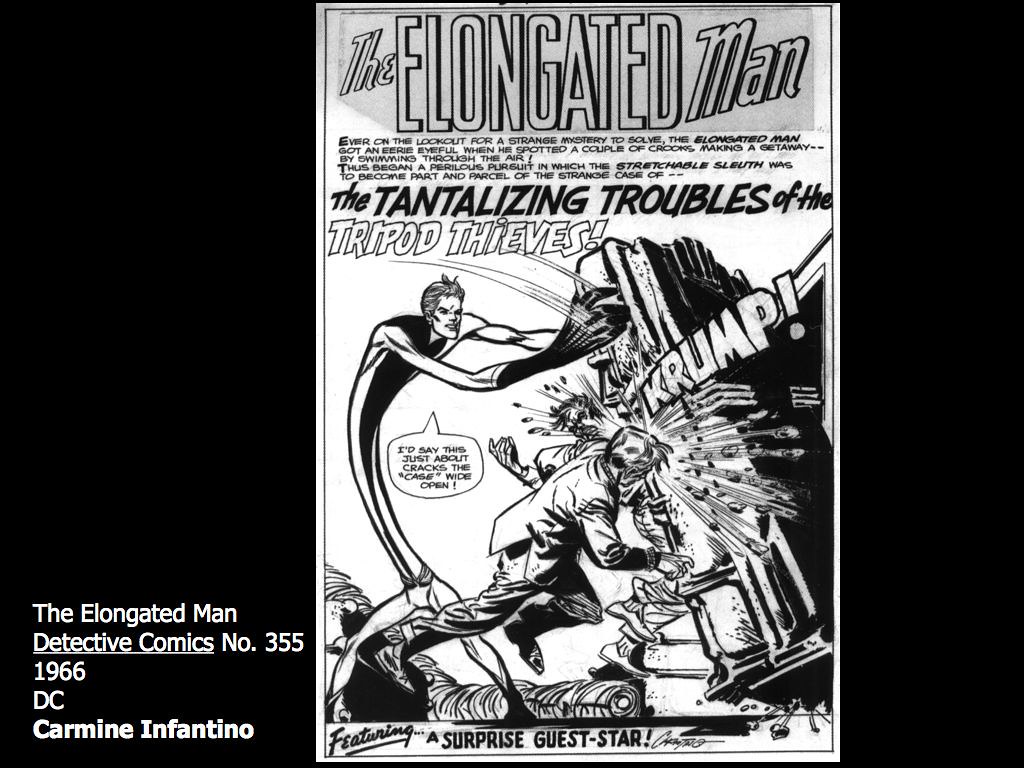The image features a black rectangle frame with a classic comic book cover entitled "The Elongated Man." The cover, created by Carmine Infantino for Detective Comics No. 355 in 1966, showcases a black-and-white illustration with varying shades of gray. Dominating the center is The Elongated Man, a peculiar superhero known for his unusually long torso, legs, and arms, demonstrating his superpowers by lifting and throwing a structure. Amidst the action, a smaller figure can be seen falling, with a speech bubble exclaiming "Crump!" The artwork includes intricately detailed text that reads, "The Tantalizing Troubles of the Tripod Thieves," along with the hero's confident declaration, "I'd say this just about cracks the case wide open." The bottom right corner notes the presence of a "surprise guest star."